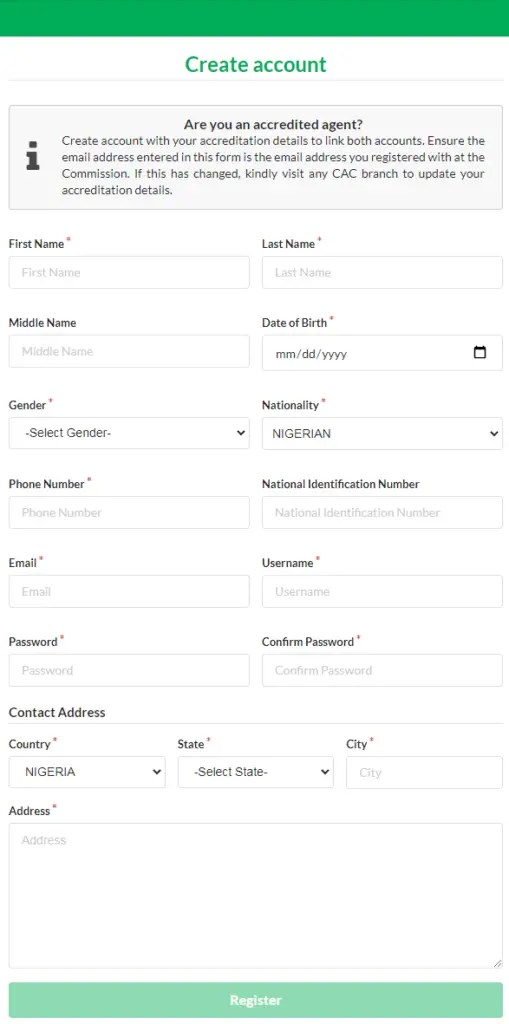The image is a tall, vertically-oriented graphic with various sections that guide the user through the process of account creation. At the very top, there is a grass green bar, followed by green lettering that reads "Create Account." Just beneath, there is a faint gray bar and a gray text box with small black letters which contain the instructions: "Are you an accredited agent? Create an account with your accreditation details to link both accounts. Ensure the email address entered in this form is the email address you registered with at the Commission. If this has changed, kindly visit any CAC branch to update your accreditation details."

Following this, there is a detailed form for the user to fill out. The form fields include:

- First Name
- Last Name
- Middle Name
- Date of Birth (MM/DD/YYYY)
- Gender
- Nationality
- Phone Number
- National Identification Number
- Email
- Username
- Password
- Confirm Password
- Contact Address (including Country, State, City, and Address)

The country field is pre-selected to "Nigeria."

At the bottom of the image, there is another grass green bar with white letters that read "Register," indicating the button for account registration. However, the button appears to be inactive. The overall layout suggests that this is a form for an official account setup, possibly related to a government or administrative process.